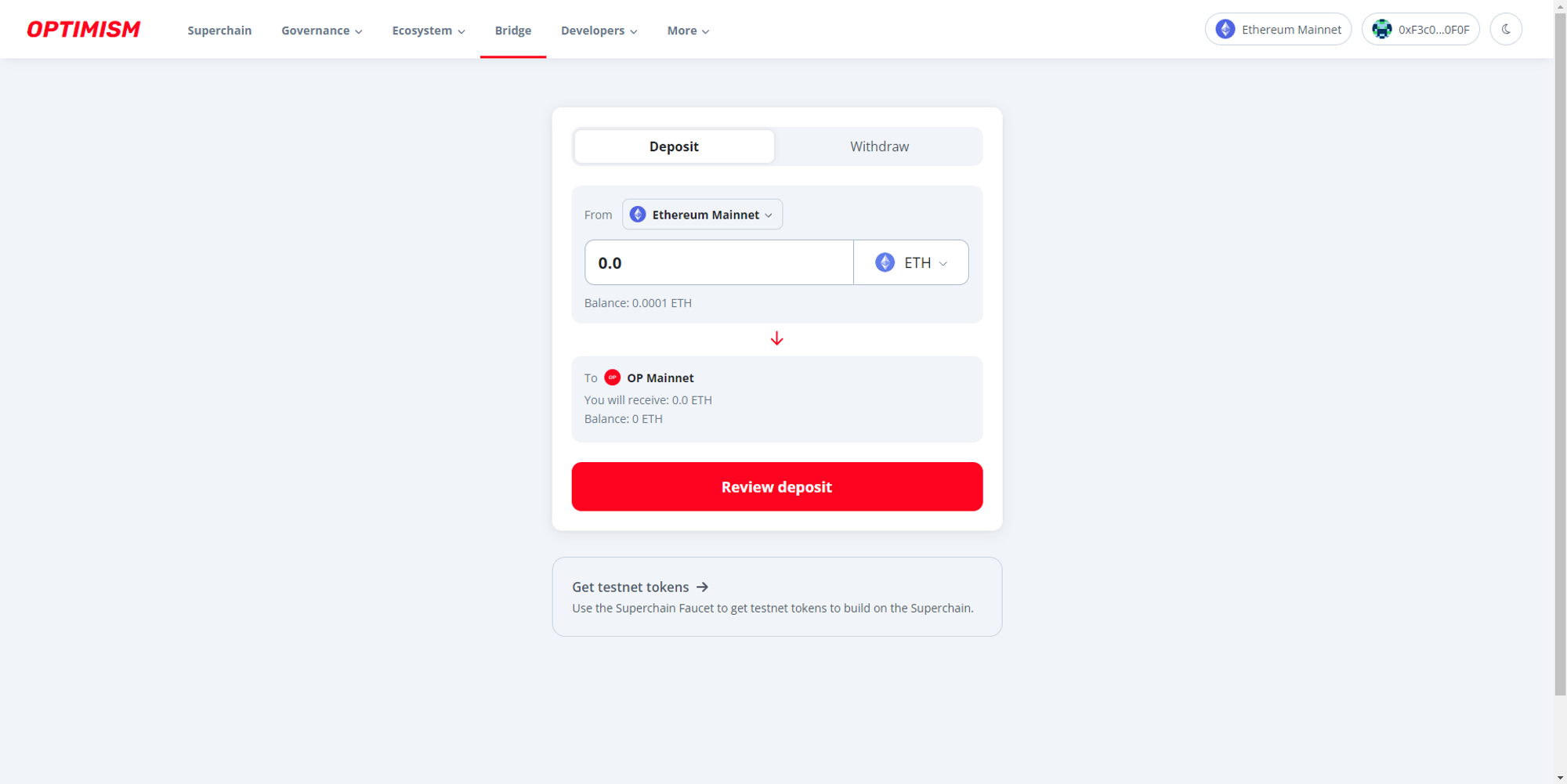This screenshot showcases the interface of a website called Optimism. In the upper left corner, the word "Optimism" is prominently displayed in red. Adjacent to it, "Bridge" is underlined in red, indicating that it has been selected.

The main feature of the screen is a large horizontal gray rectangle. Within this rectangle, there is a smaller white-bordered square at the top that contains the text "Deposit and Withdrawal." The "Deposit" button is highlighted in white, suggesting it has been selected. Below this, the text reads "From Ethereum Mainnet," accompanied by a box where users can input an amount. This box also shows the current balance and includes a red downward-pointing arrow.

Further down, it says "To OP Mainnet," displaying "You will receive 0.0 ETH, balance 0 ETH." At the bottom of the gray rectangle, a large red button stretches across the width, marked "Review Deposit" in white text.

At the very bottom of the screenshot, there's a smaller, rounded gray rectangle with the text "Get Testnet Tokens" followed by a right arrow. It instructs users to "Use the superchain faucet to get testnet tokens to build on the superchain."

Overall, this detailed interface provides a clear indication of the deposit process from Ethereum Mainnet to OP Mainnet, along with options for obtaining testnet tokens for development purposes.